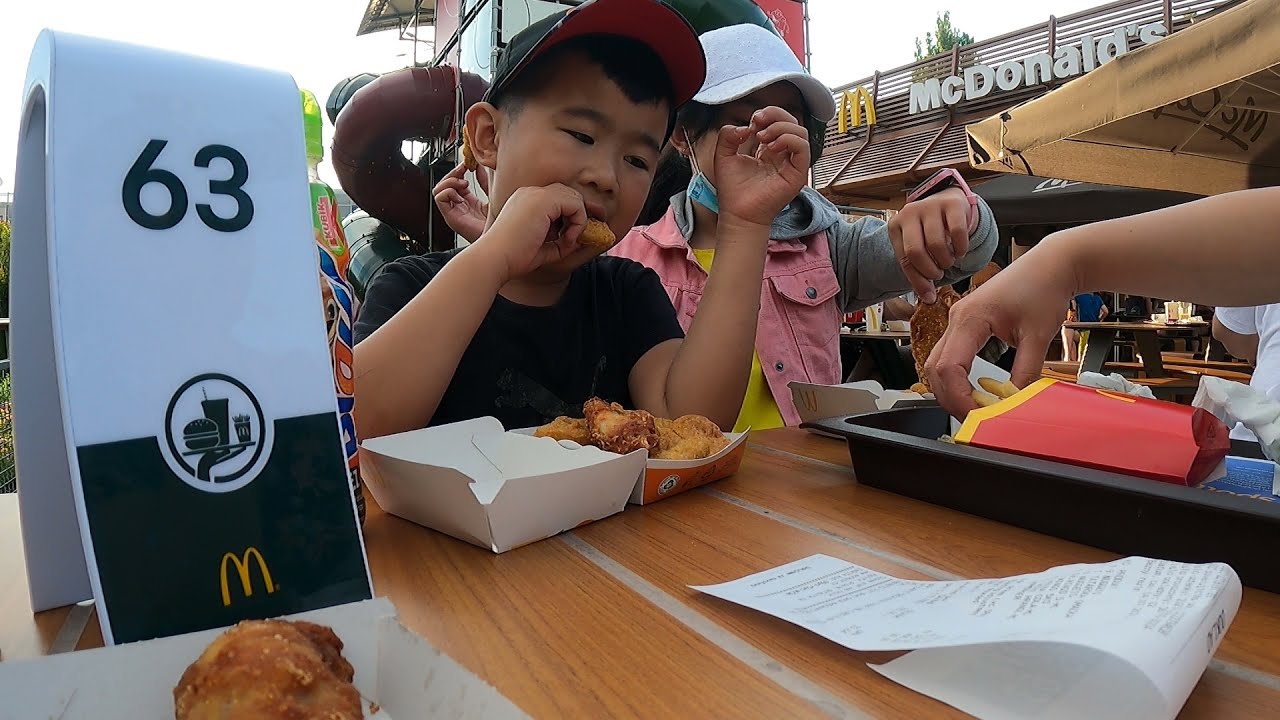In this lively outdoor scene at McDonald's, a young boy, around seven or eight years old, is enjoying chicken nuggets while wearing a black and red baseball cap and a black t-shirt. His short black hair peeks out from under his cap. To his right is a girl in a pink jacket and blue hat, also seemingly engrossed in her meal. A piece of the table marker sign displaying the number 63 and a McDonald's M logo is visible on the left side of the image. A folded white receipt lies on the table's right-hand corner. Adding to the quintessential McDonald's experience, a red box of fries sits on a tray to the right with someone's hand reaching in to grab some. In the background, the iconic McDonald's sign with the golden arches and the word "McDonald's" is clearly visible, alongside a light brown McCafe umbrella, hinting at a pleasant, sunny day. Additional picnic tables and a glimpse of the McDonald's playground complete this vibrant setting.